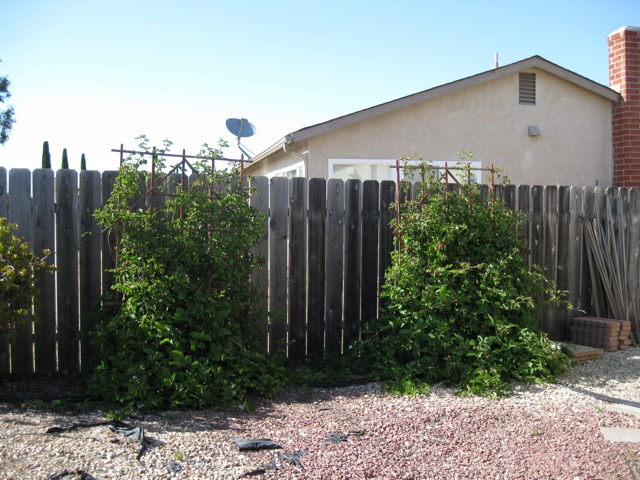This photograph captures a detailed scene of someone's backyard, featuring a ground covered in a mix of light reddish-brown and whitish stones with a hint of black tarp peeking out on the left side. Dominating the scene is a tall, weathered wooden fence with grayed planks, standing straight across the middle. In front of this fence, two dark brown wooden trellises support lush green vines, adding a touch of nature to the otherwise man-made setting. Behind the fence, towards the upper right, stands a light yellow-colored house with a slanted roof. The house features a red brick chimney on its right side and a satellite dish on the left side of the roof. Above, the sky transitions from a light blue at the top to whitish near the horizon on the lower left side.